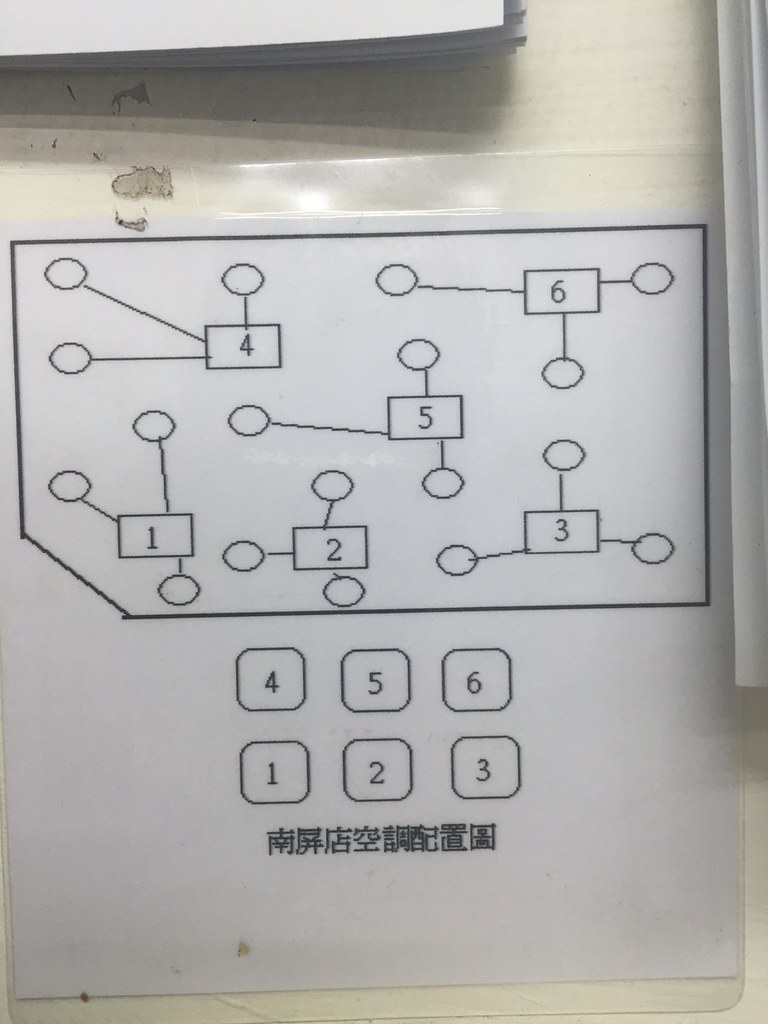A laminated white card is prominently displayed against a painted cream-colored surface. The card, encased in protective plastic, features what appears to be Chinese text in a single line at the bottom. This text, comprised of ideograms, suggests the card's origin or instructions. Above the text are six rounded rectangles arranged in two rows of three. The bottom row is sequentially labeled 1, 2, 3, while the top row is labeled 4, 5, 6.

Positioned above these labeled rectangles is a detailed diagram contained within a black-rimmed rectangle that has one corner cut off, reminiscent of the shape of an old holograph card. Within this diagram, six boxes are visibly labeled 1 through 6. Each of these boxes features three lines radiating outward, each terminating in a small circle. The pattern of these lines and circles varies in length and direction among the boxes, creating unique configurations within each numbered section.

The card itself is pristine white with a high-gloss laminate finish, though it has some adhesive residue visible at the top and bottom edges, suggesting it may have been previously affixed to another surface. This residue adds a subtle texture contrast to the otherwise smooth laminated surface.